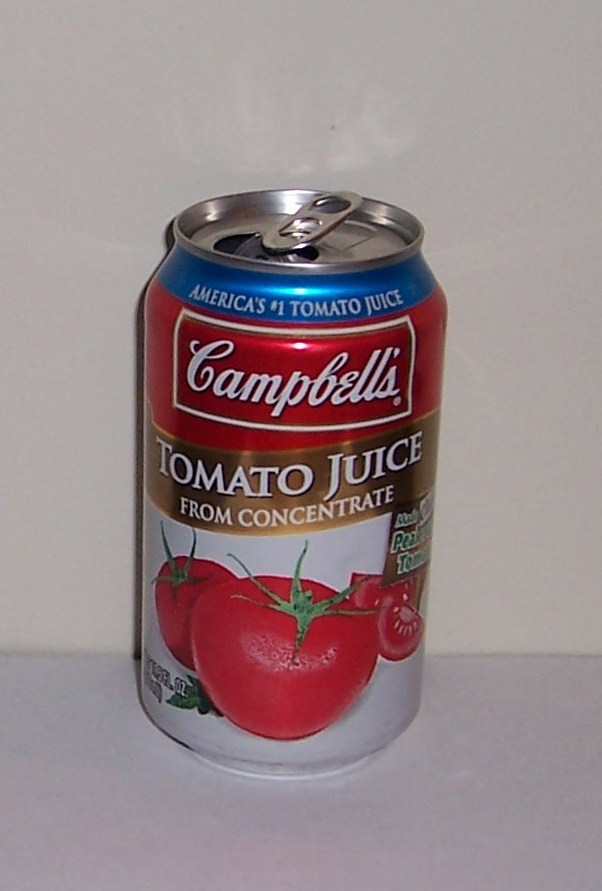This photograph showcases a Campbell's tomato juice can, embodying the classic Campbell's signature design, with a distinctive red background and white lettering. The can is produced entirely from aluminum with the iconic label elements printed directly onto the surface, rather than a paper label. It features a pop-top tab for easy opening.

Prominently displayed underneath the "Campbell's" logo are the words "Tomato Juice from Concentrate." The design includes the imagery of two whole tomatoes, along with several sliced tomato pieces to the right. Positioned above the sliced tomatoes, partially obscured text likely reads "Peak Freshness Tomatoes," though only the words "Peak" and "Tom" are fully visible. On the bottom left corner of the can, there is an indication of the can's volume, though the specific ounce measurement is not clearly visible. The can appears to be of a standard size similar to that of a typical soda or juice container.